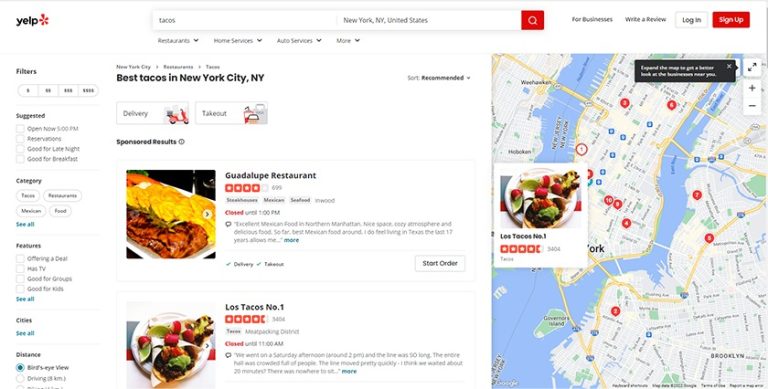A screenshot displays a Yelp search page against a white background. At the top, the search bar contains the query, "tacos New York, New York, United States." Next to the search bar is a red square with a magnifying glass icon, indicating the search function. Below this, options for "For Businesses," "Write a Review," and "Log In" are presented in a white rectangle, while "Sign Up" appears in a red rectangle.

To the right of the search results, a map is visible displaying numerous business logos. The first search result shows "Los Tacos No. 1," a highly-rated taco spot in New York City, lauded as the best for tacos in the area. It features a prominent status showing "closed until 11 a.m.," along with options for delivery and takeout. This establishment has received 4.5 stars from reviewers.

Another highlighted business is "Guadalupe Restaurant," which has earned four stars and also offers delivery and takeout. This restaurant is marked as "closed until 1 p.m." and includes a "Start Order" button in a white rectangle for easy online ordering.